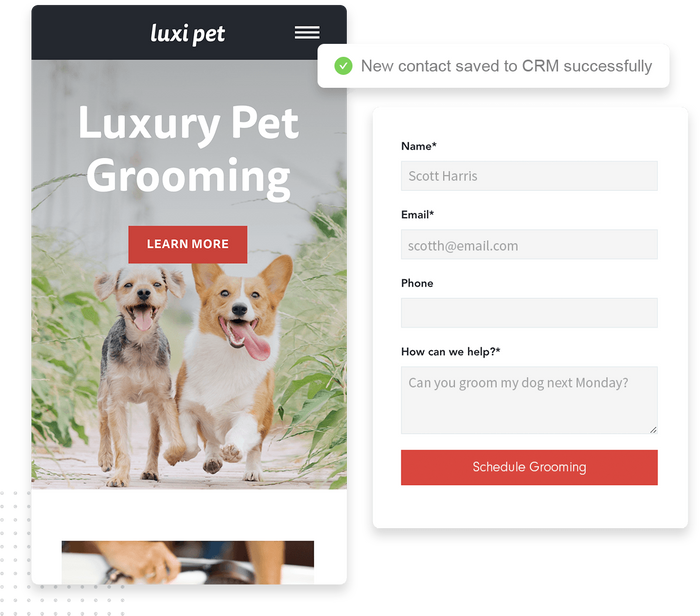This image appears to depict a screenshot from a mobile application or a mobile webpage designed for a luxury pet grooming service called Luxy Pet. The top of the display features a black bar with the text "Luxy Pet" written in white. Below this, there is an artistic rendition of two dogs running side by side, accompanied by the phrase "Luxury Pet Grooming." A red rectangle with the text "Learn More" invites users to explore further.

To the right of this illustration is a prominent notification in a white rectangle, which reads "New Contact Saved to CRM Successfully," featuring a solid green circle with a check mark symbolizing a completed action.

Below this notification, there are four input fields. The first field, labeled "Name" with an asterisk denoting it as a required field, is filled in with "Scott Harris." The second field is labeled "Email," also marked with an asterisk, contains "scott at email dot com." The third field, "Phone," remains empty. The fourth field, titled "How Can We Help?" with an asterisk, has a larger text box filled with the query, "Can You Groom My Dog Next Monday?" At the bottom of this section is a red rectangle button with white text reading "Schedule Grooming."

In the uncropped bottom portion of the image, there is a partial picture showing hands engaged in an unidentified activity, but the image is cut off, making it unclear what the hands are doing.